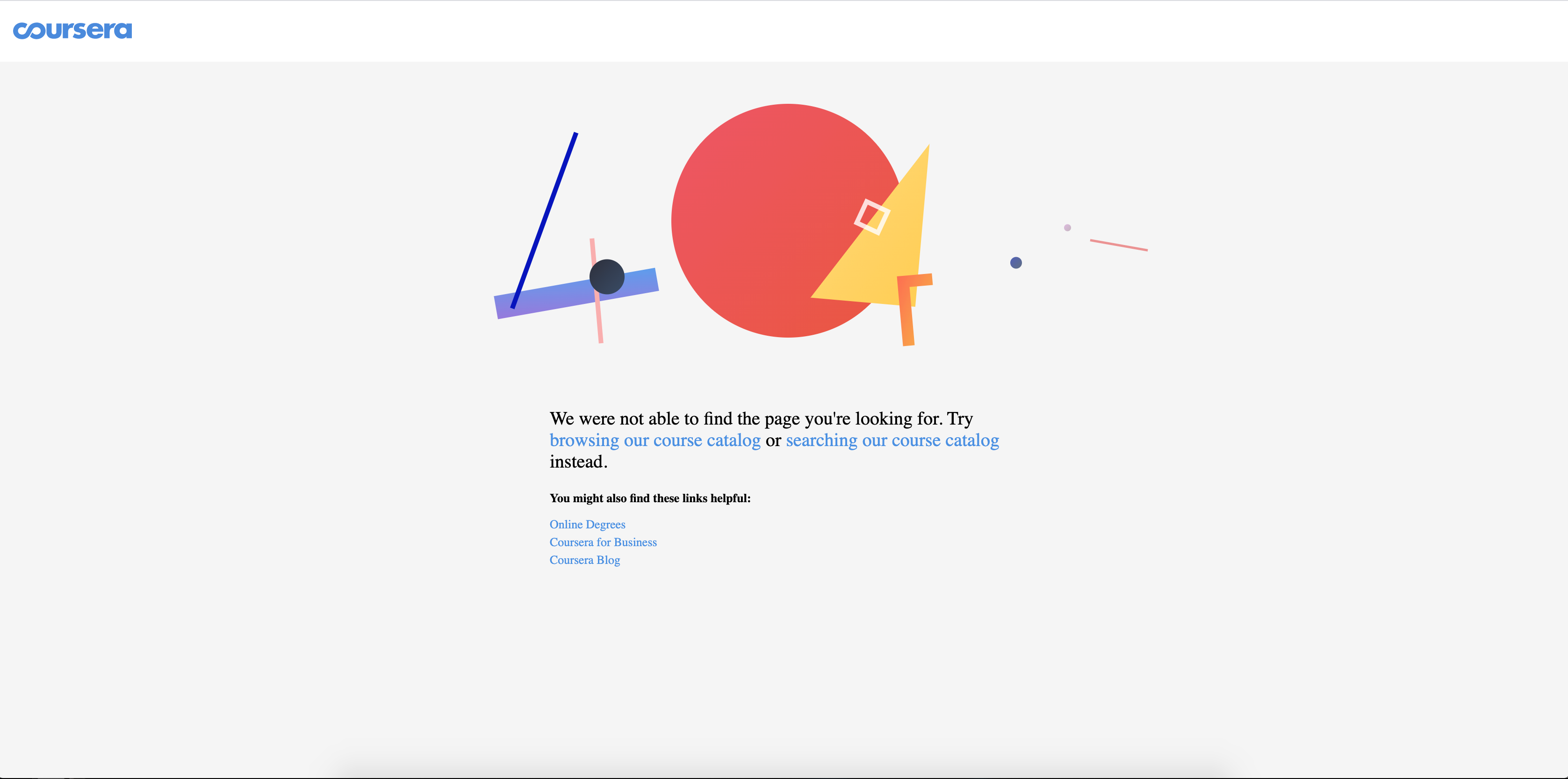The image depicts an error page on the Coursera website. The Coursera logo, written in blue, is located in the upper left-hand corner of the webpage. The main body of the page features a large gray box. Positioned prominently above the text within this box is an eclectic mix of colorful shapes: a large red circle, what appears to be a skateboard adorned with a pink stick and a circle, a yellow triangle, a small white box, an upside-down orange "L," a blue dot, a small purple dot, and a tiny red stick.

Below these shapes, the text in black reads, "We were not able to find the page you're looking for." The message suggests browsing or searching the course catalog, with both options highlighted in blue. Additionally, there's a note indicating, "You might also find the following links helpful," though the text is quite small and hard to read. Beneath this note, there are three links, also written in blue. This image essentially informs the user that the webpage they attempted to access could not be found, indicating an error.